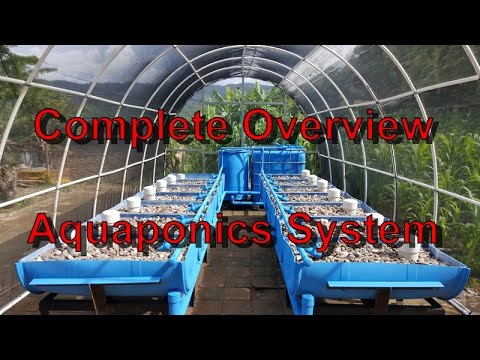In this low-resolution, indoor photograph resembling a still frame from a video, we see an aquaponics system inside a dome-shaped greenhouse. The structure is built from a clear plastic material or glass panels supported by a silver-colored metal framework, with white tubing bordering each panel. This image, framed by black letterbox bars on the top and bottom, is taken from the vantage point of someone standing inside the greenhouse, looking down a central aisle flanked by long rows of aquaponics bins. 

The bins, made from blue plastic drums cut in half, are lined with gray rocks and white PVC pipes, presumably where plants will grow. These bins are situated on either side of the aisle, which is paved either with reddish-brown brick tiles or wooden planks. At the end of the aisle, several large blue vats or tubs, encircled by blue railings, presumably serve as water reservoirs for the system. 

A fluorescent light fixture is visible in the top right corner of the image, adding to the artificial lighting. To the right, there are green plants, while the left side shows patches of brown soil. The greenhouse's domed roof curves elegantly towards the top, revealing a gray, overcast sky in the top left corner. Overlaid in bold red text with a black outline, the image is titled "Complete Overview Aquaponics System."